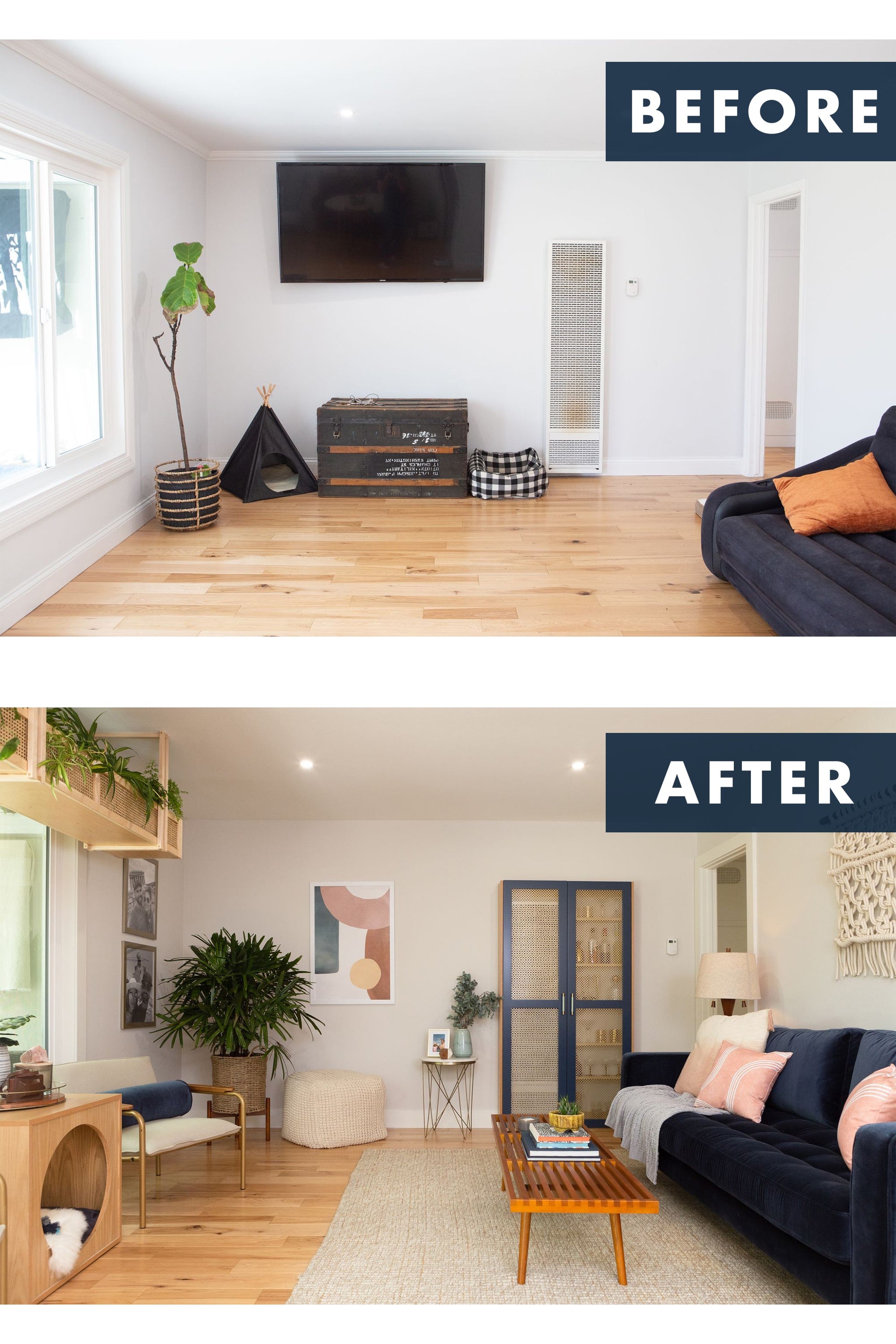The image consists of two photos of the same room demonstrating a before-and-after transformation. In the "before" image, which is marked in white letters on the right-hand side against a dark background, the room features plain white walls, a window on the left with minimal attachments, a flat-screen TV mounted on the wall, a sparse floor plant, a partial view of a dark couch on the right side with an orange pillow, and light plank flooring. There's also a trunk visible on the far side under the window.

In the "after" image, labeled similarly with "after" in white letters on a blue background, the room has undergone significant changes. The walls are painted gray, and the decor is more elaborate. The TV has been replaced with a piece of framed art. Above the window, a shelf has been installed with hanging plants, while a nicer, fuller plant in a woven basket replaces the initial sparse one. The floor is now adorned with a smooth white rug. A small chair is substituted by a full, comfy blue sofa adorned with multiple throw pillows. There is a wooden coffee table placed in front of the sofa. Additional enhancements include a seating bench by the window, a new coffee table with wood slats and feet, and a lamp beyond the couch, making the room appear cozier and more inviting.